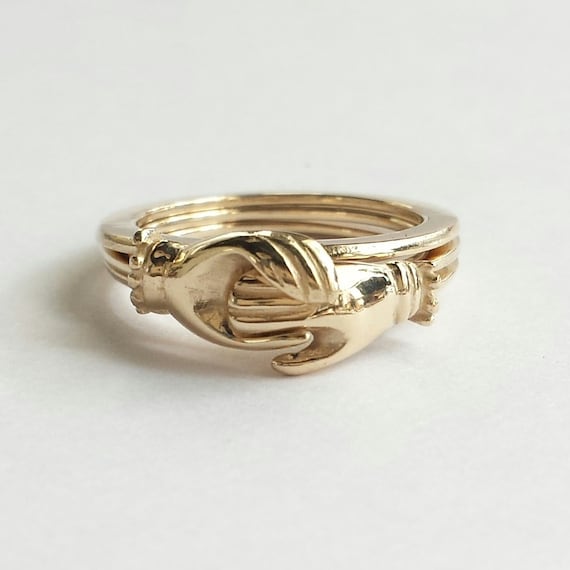This photograph showcases a close-up of a simple yet symbolically rich gold ring set against an off-white, beige-colored background, illuminated from above. The ring features two hands intricately clasping each other, forming the focal point at the top, where a gem might typically sit. The hands have a stylized fringe, adding a unique touch to the design, and the ring’s underside includes distinct ridges. The bright, reflective gold surface indicates its shiny, polished finish. The image captures subtle shadows beneath the ring, emphasizing the central composition and the joined bands at the back. The ring's design, evoking a sense of unity and relationship, suggests it could be a meaningful token, possibly symbolizing love or marriage.